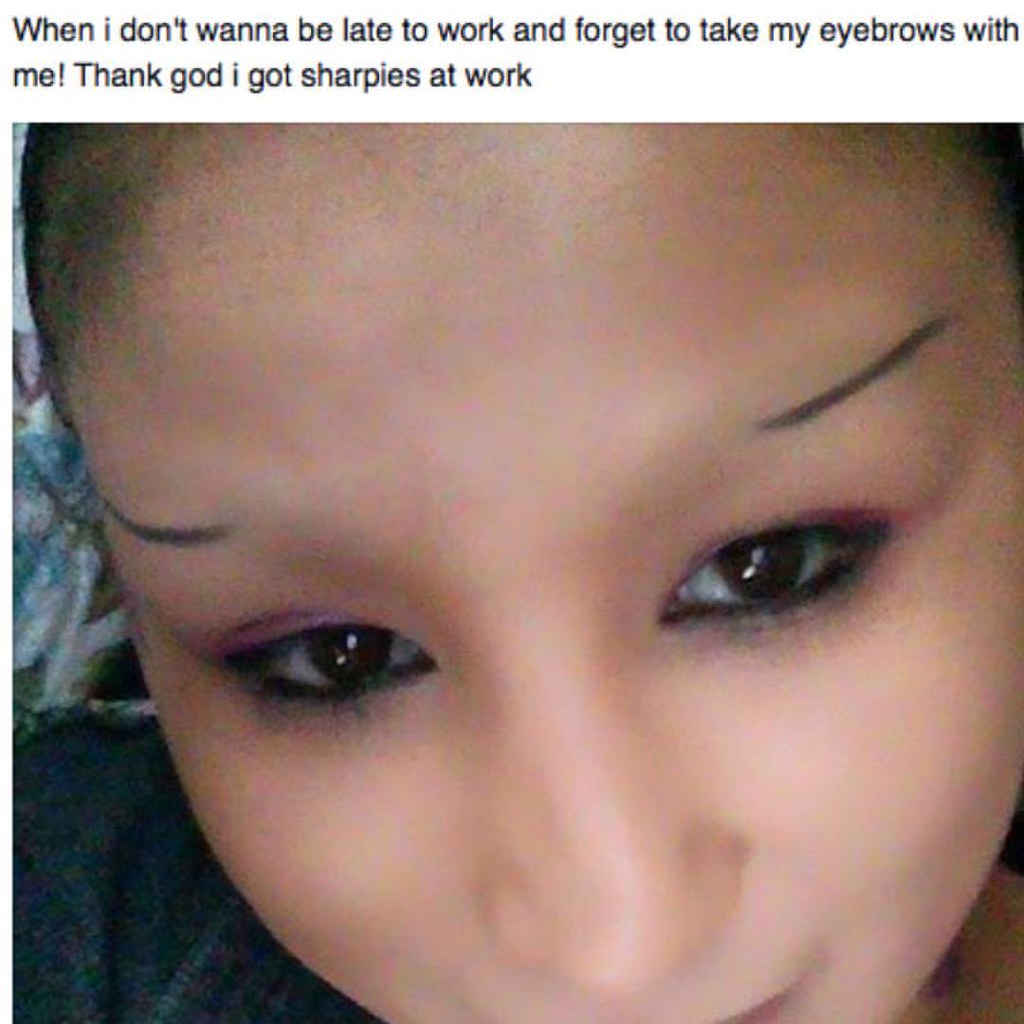The image is a close-up shot of a young woman's face, with the focal point being her expressive, dark brown eyes. Her smooth, medium-toned complexion gives her face a serene appearance. Notably, she lacks both hair and eyebrows, suggesting she may be undergoing some form of treatment, with just a hint of stubble on her head indicating regrowth. Her eyebrows are represented by two thin, short lines of dark makeup. She is wearing black mascara and subtle pink eyeshadow, which accentuates her eyes further. The woman is dressed in a dark gray sweater, and behind her is a pillow adorned with white, blue, and green patterns. A light source from above highlights the top of her head, creating a slight shine. Additional context is provided by text above her, humorously noting, "When I don't want to be late to work and forget to take my eyebrows with me, thank God I got Sharpies at work." She gazes directly into the camera with a composed expression.